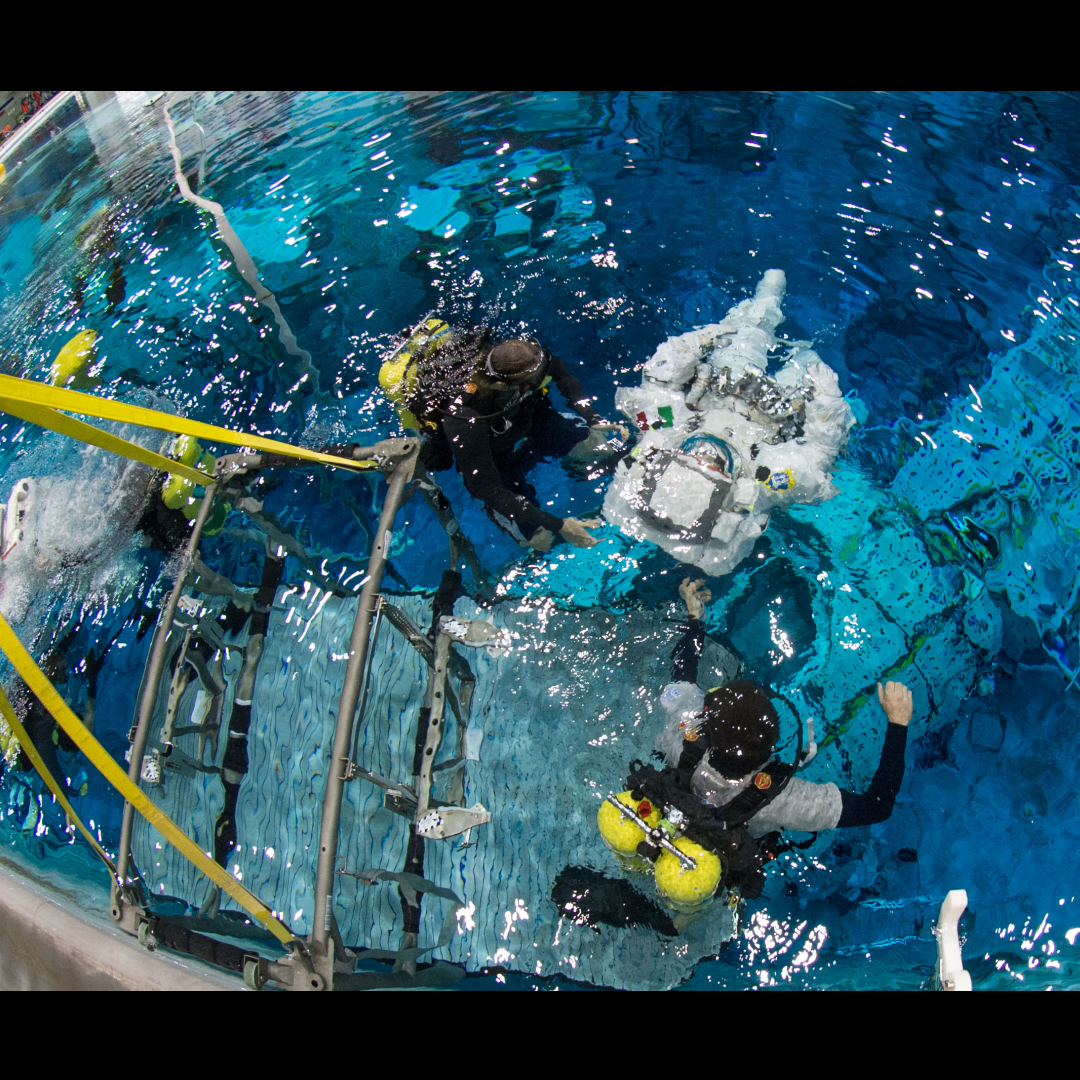This photograph captures a vivid underwater scene in a circular, bright blue pool, where four individuals are engaged in an activity. Three of these individuals are prominently positioned in the center, while a fourth person is partially visible to the left. Central to the image is a person clad in a white astronaut suit, surrounded by two scuba divers. The diver to the left of the astronaut is outfitted in black with a gray t-shirt over the scuba suit, and the diver to the right is wearing a full black scuba suit. Both scuba divers have yellow oxygen tanks strapped to their backs. They appear to be examining a white object submerged at the bottom of the pool, which resembles a plane or spacecraft. On the left side of the frame, four yellow straps attached to a gray metal cage or basket are visible, seemingly suspended in the water. The pool is illuminated by artificial lights, creating a reflective surface and illuminating the submerged machinery barely visible at the pool's base.